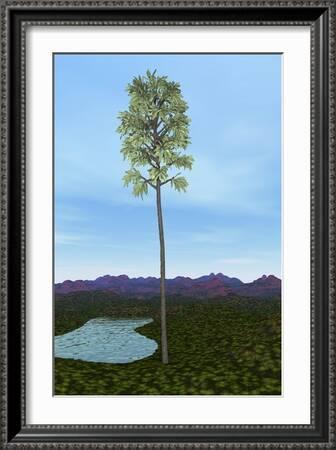This caption provides a detailed description of the framed image, emphasizing the repeated details described by multiple people:

Framed within a black picture frame with intricate detailing and a white mat border, the artwork captures a surreal yet evocative scene. At its center stands an extraordinarily tall and thin tree, bearing a striking resemblance to a palm tree. The tree's trunk, extending to nearly two-thirds or more of the tree's height, is devoid of branches until the very top, where a small cluster of branches sprouts, adorned with green leaves. Surrounding the tree is a green field with vegetation, and to the left of the tree, there's a small, calm pond. In the background, a range of mountains, varying from purplish to reddish hues, stretches across the horizon, under a light blue sky with faint clouds. The scene evokes a sense of otherworldly tranquility, enhanced by its painterly quality, making it ambiguous whether it is a photograph or a painting.